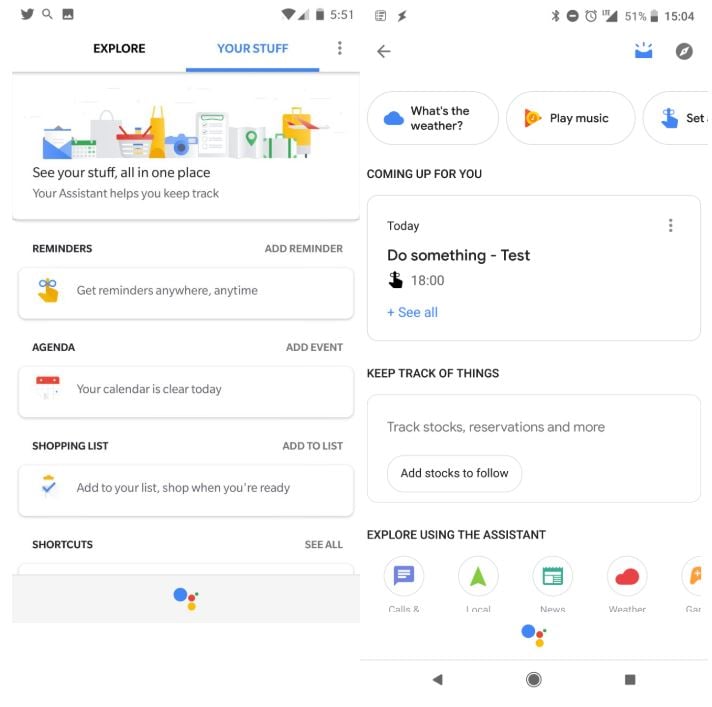This diptych features two screenshots of mobile applications, both presenting a white background with dark gray icons situated in the top left and top right corners. 

In the left screenshot, the header contains the words "Explore" in black text on the left, followed by "Your stuff" in blue text accompanied by a blue underline, and three medium gray vertically stacked dots to the right. Below this header section is a white rectangular tile with a light gray shadow above and below, showcasing a variety of colorful clipart-style objects arranged horizontally. Underneath this tile, black left-justified text reads "See your stuff all in one place," followed by light gray text stating, "Your Assistant helps you keep track." Below this main tile, outside of its boundary, you'll find the black text "Reminders" on the left, with dark gray text "Add reminder" on the right. Another shorter tile appears beneath, featuring a colorful icon of a cartoon hand with a blue bow tied around its finger and adjacent light gray text reading "Get reminders anywhere, anytime." Further down, the next tile is labeled "Agenda," containing an "Add event" option to its upper right. This tile includes an icon of a calendar with a red bar across the top and the text, "Your calendar is clear today." The final tile at the bottom is labeled "Shopping list."

In the right screenshot, the top left corner houses a medium gray left-pointing arrow, while the top right corner contains two icons: a blue file container with three blue lines radiating outward and a dark gray compass icon to its right. This layout and the concise but clear placement of each element guide the user effortlessly through the application's functions.